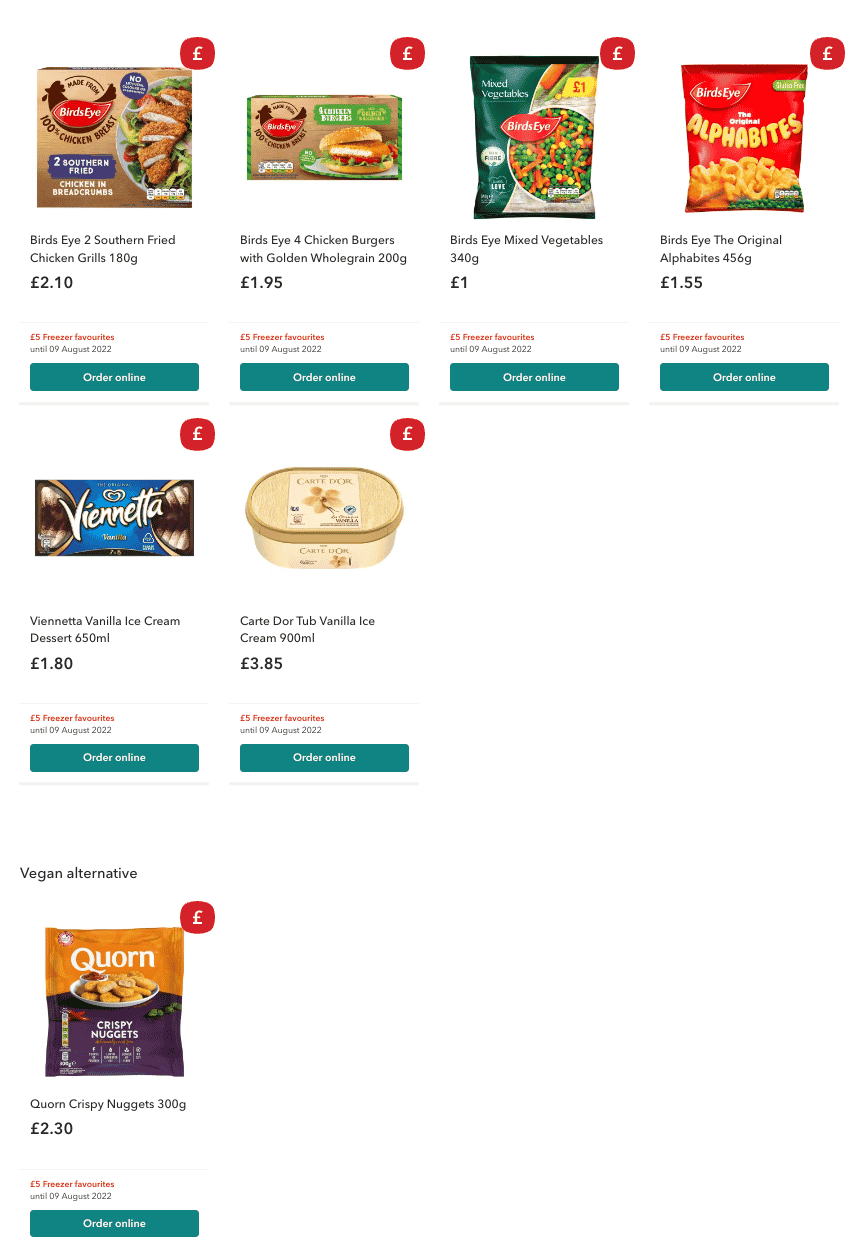This screenshot captures the interface of an online grocery delivery service. The backdrop is a minimalist white, ensuring the focus remains on the various food items displayed. Featured prominently are seven frozen food products, each accompanied by a corresponding image. The items listed include:

1. Bird's Eye Southern Fried Chicken
2. Bird's Eye Chicken Burgers
3. Bird's Eye Mixed Vegetables
4. Bird's Eye Original Alphabet Potato Shapes
5. Vienetta Vanilla Ice Cream Cake
6. An unspecified carton of ice cream
7. Quorn Vegan Crispy Nuggets

Each product is provided with detailed information, including pricing displayed in pounds, product weight, and a visually distinct "Order Online" button in a muted green hue. This straightforward yet effective layout underscores its purpose as a convenient click-and-deliver grocery service.